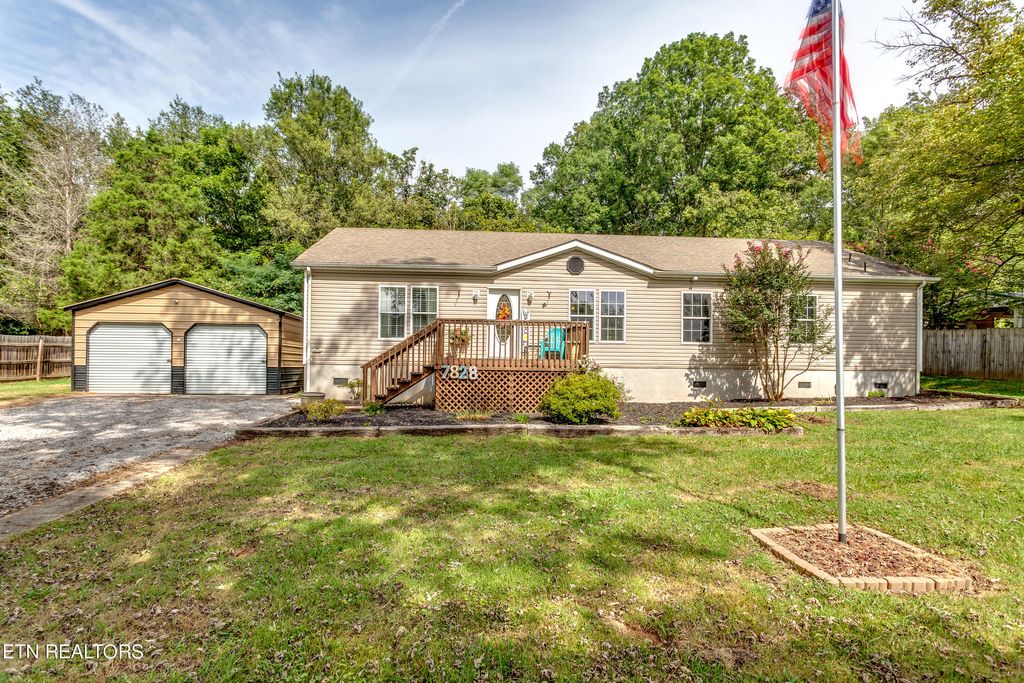This image features the front view of a large, single-story house with a mobile home-like appearance. The house is tan with yellowish-beige paneling and a brown roof, and it is adorned with the address number "7828" in silver, light brown, blue, and grayish-pink. Leading up to the front entrance are brown steps. Prominently displayed in the grassy front yard is a flagpole with a large American flag flowing in the wind, surrounded by a small mulch area. The yard includes green grass interspersed with patches of brown, a small tree against the house, and some bushes. The house's façade features six windows and a white front door, with four additional windows along the side. To the left of the house, a two-door garage or shed, also tan with a brown roof, is partially enclosed by a wooden fence that surrounds the entire property. ETN Realtors is indicated in the bottom left-hand corner of the image. The background is enriched with several large, green, and lush trees.